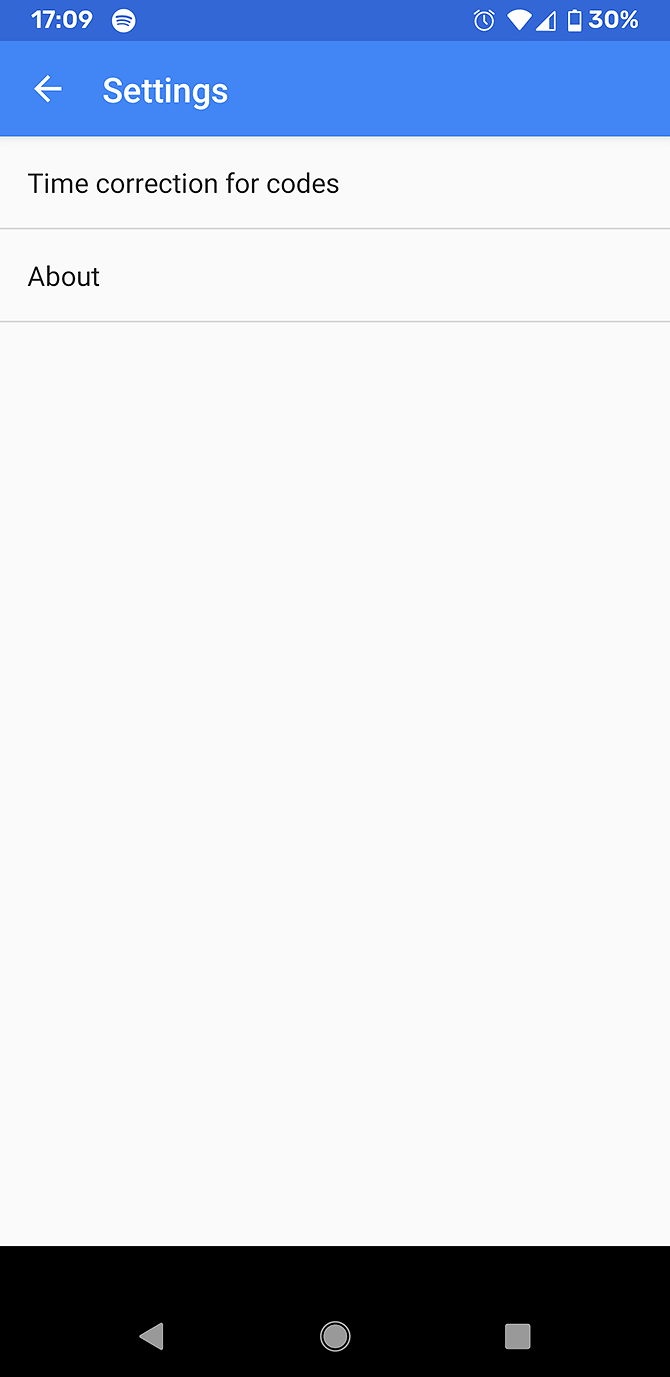The image is a screenshot of the settings page on a mobile device. At the very top of the screen, there's a dark blue status bar. In white text on the left, it reads "17:09" indicating the time. To the right of the time, there's a Spotify icon, followed by gaps that accommodate various phone status icons, including an alarm icon, a Wi-Fi signal indicator, a signal strength marker showing three out of four bars, and a battery icon indicating a 30% charge, with "30%" displayed next to it.

Below the status bar is a slightly lighter blue navigation bar. On the left, in white text, it says "Settings" accompanied by a left-pointing arrow. 

The main content area of the screenshot features a light gray background. The first item listed is "Time correction for codes," rendered in black sentence-case text. Beneath this, there's a thin gray divider line. The next item on the list is "About," also in black text with a capitalized first letter, followed by another identical gray divider line. The rest of the main section is empty.

At the very bottom of the image, there is a black navigation bar containing three classic Android navigation icons: a left-pointing triangle, a circle in the center, and a square on the right.